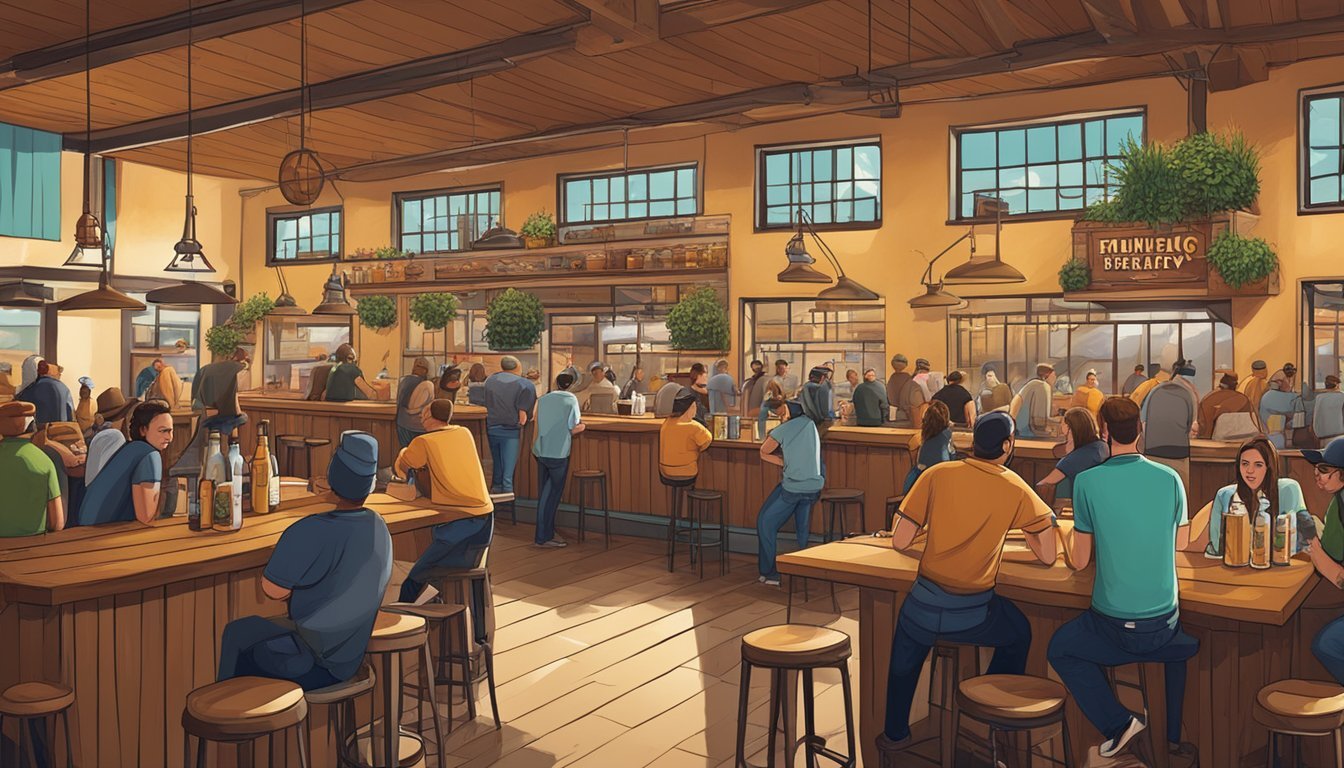This image is a detailed, computer-generated drawing of a vibrant restaurant and bar, characterized by its extensive use of brown wood throughout. The room is rectangular and features a high ceiling adorned with wooden planks and large, criss-crossing dark wooden beams. Numerous hanging lights illuminate the space. The walls are a warm orangish-brown stucco, complemented by green plants hanging and positioned against the back wall. 

A row of windows with grids and brown frames spans the top portion of the back wall, and another set of high ground-level windows integrates with the layout. In the back left, a blue curtain is visible. The interior is bustling with activity, depicting mostly fair-skinned patrons who wear blue jeans, yellow shirts, blue shirts, and some cowboy hats. Men and women, some with brown hair, are seated on high-top wooden stools or at rectangular wooden tables with round stools, enjoying their meals and drinks that appear to be alcohol in brown liquid jars and bottles. 

Amid the lively crowd, people are either sitting, standing, or behind the bar serving drinks. There are light fixtures hanging from the ceiling, adding to the cozy atmosphere. A prominent wooden countertop runs along the back, with several stools placed in front of it where more patrons are gathered. Above, a wooden sign with yellow text, partially obscured and unreadable, hangs, accompanied by green plants. Overall, the image portrays a lively, wood-paneled restaurant and bar filled with cheerful people against a rich backdrop of warm tones and greenery.